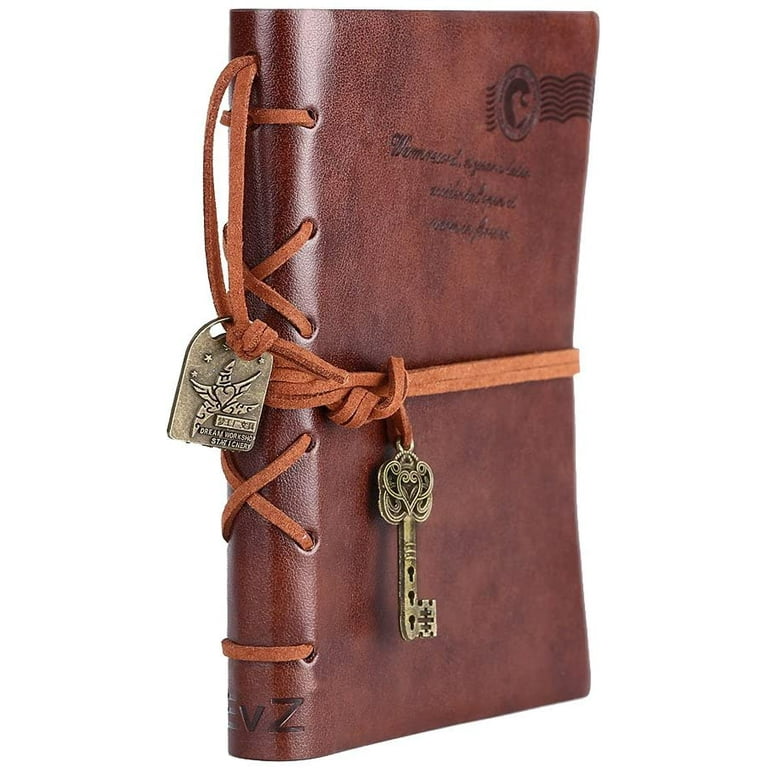This is a high-quality, professional photograph of a vintage-style, leather-bound journal. The journal is encased in a reddish-brown, almost maroon-brown leather, which gives it a rustic and luxurious appearance. Its binding is uniquely crafted with a thin, braided leather cord that is woven through punched holes along the spine, securing the journal closed.

The cover features some black, cursive text that is faded and difficult to read, suggesting it might be an embossed or stamped design. Additionally, there is a black logo or emblem at the top of the cover that adds to its antique charm.

Attached to the binding is a delicate, old-fashioned metal key and a small metal charm, possibly in the shape of a star or butterfly, adding to the journal's whimsical and mysterious appeal. The color palette of the image includes variations of black, white, gray, silver, light brown, and dark reddish-brown, making it visually striking against the white background, reminiscent of images found on high-quality, professional websites like Google Images.